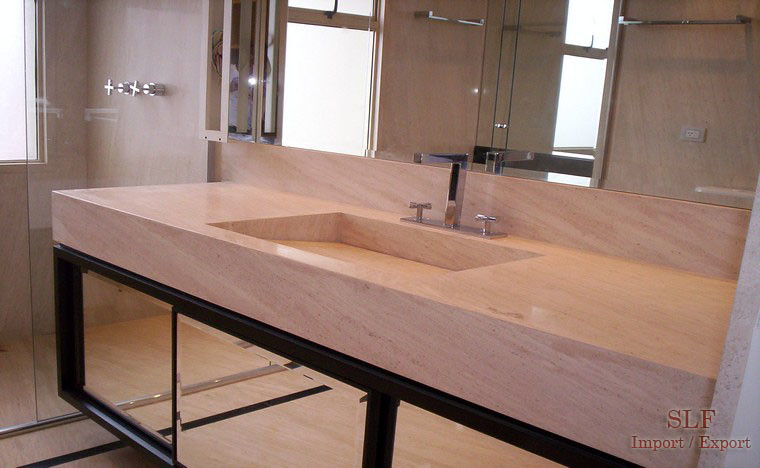This landscape-oriented photograph captures the pristine interior of a modern bathroom. The room features a light coral marble aesthetic, creating a warm and inviting atmosphere. The sleek coral-colored sink is characterized by an elegant cut-out design, and beneath it lie three sliding mirrored panels that offer additional storage and reflectivity. Above the sink, large mirrors span the wall, amplifying the sense of space and reflecting various elements of the bathroom. To the left, a clear glass shower enclosure with sliding doors stands in front of a frosted window, allowing diffused daylight to softly illuminate the space. The fittings, including faucets and shower fixtures, are all finished in polished silver, adding a touch of sophistication to the overall design.